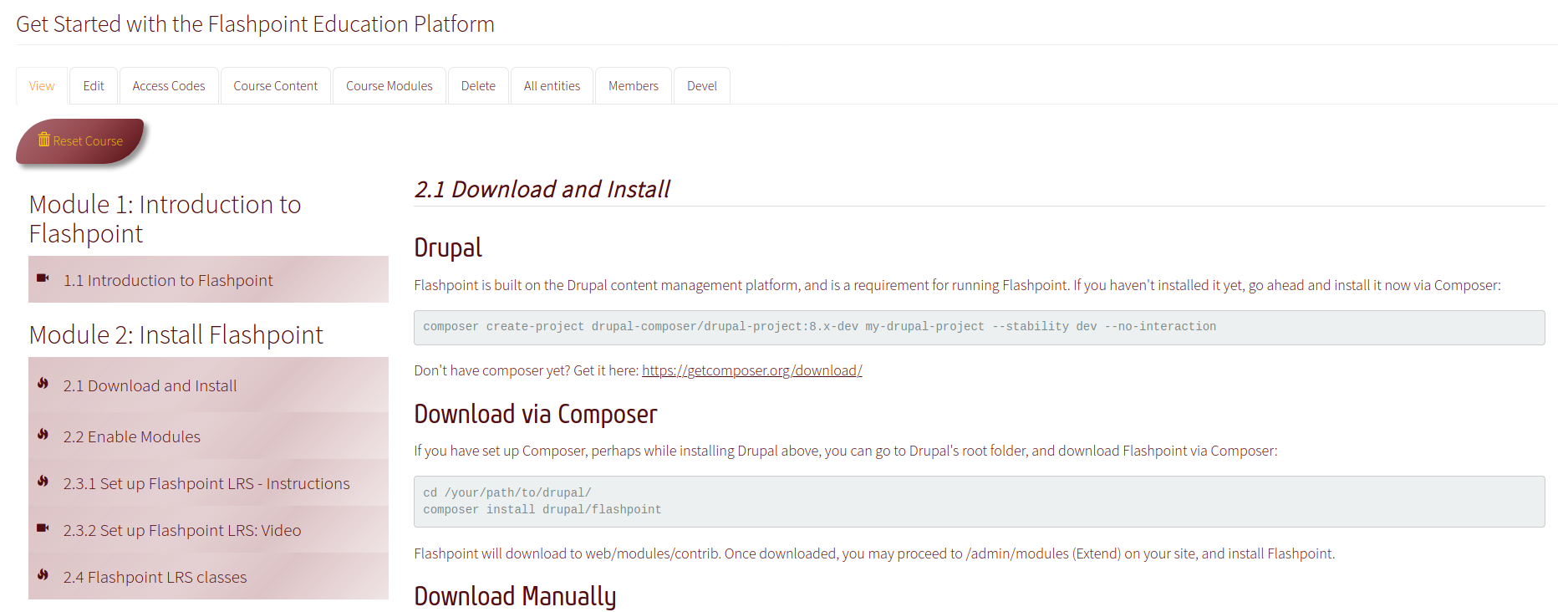In the screenshot, the image displays the interface of what appears to be an educational platform website called "Flashpoint Education Platform." Dominating the upper left-hand corner is the title, "Get Started with Flashpoint Education Platform," presented in a dark reddish text color. Directly beneath this title are rectangular menu buttons labeled: View, Edit, Access Codes, Course Content, Course Modules, Delete, All Entries, Members, and Development.

Further down, there is a prominent red button labeled "Start Course." The website then transitions into a structured single-column layout depicting the course modules. The sequence starts with "Module 1: Introduction to Flashpoint," followed by "Module 2: Install Flashpoint." Each module is outlined in an organized manner, providing categories such as: Introduction to Flashpoint, Install Flashpoint, etc.

To the right of this module listing, additional subtopics under Module 2 are displayed, including "2.1: Download and Install," "Drupal Download via Composer," and "Download Manually." This structured layout indicates a clear, step-by-step approach designed to guide the user through the course content systematically.